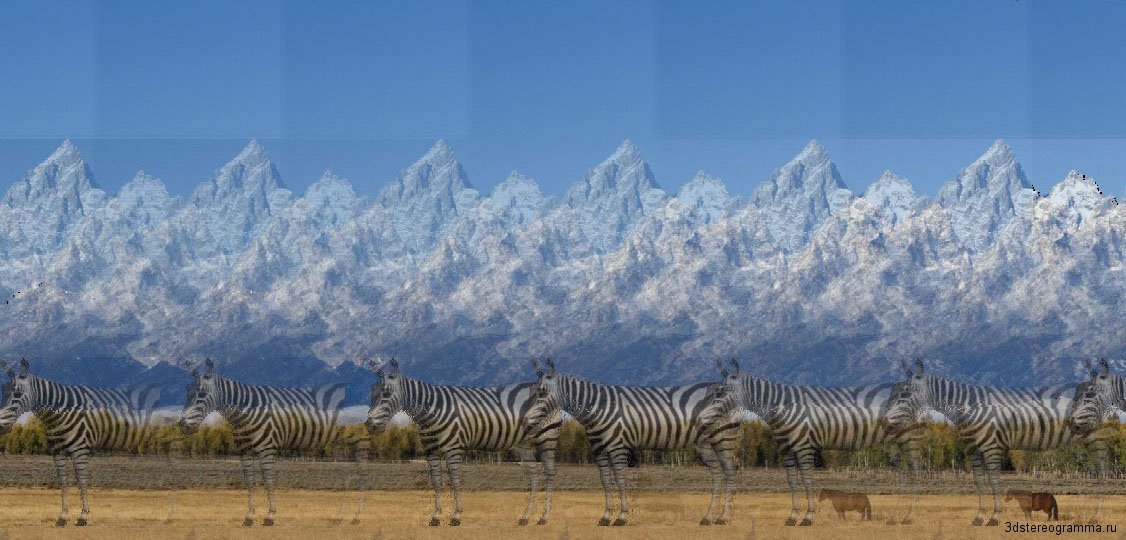This detailed panoramic image is a striking example of an optical illusion. Horizontally oriented in a rectangular frame, the scene showcases a surreal composition with several elements duplicated across the landscape to create a mesmerizing effect. The foreground features a computer-generated zebra in profile, its left side facing the viewer. The zebra appears to be superimposed over itself multiple times, creating a seamless pattern of seven and a bit repeated images. 

Before the repeating zebras is a plane of brownish-tan grass, split horizontally with a lighter yellow foreground and a darker gray background. Above this grass plane, there is a skyline of trees on the horizon that adds depth to the scene. The backdrop features a series of white-peaked, snow-capped mountains, each mountain replicated to appear as if copy-pasted, forming a continuous and repetitive pattern across the background. The sky is a vibrant cerulean blue, with no clouds in sight, and it too is constructed from replicated blocks to mirror the rest of the image's tiled nature.

On the very bottom left corner, the image includes a duplicated logo of a horse, with a website address beneath it, reading "3dstereogramma.ru." This contributes to the overall feel of an art piece designed with technical precision, likely intended for a poster or digital publication. The detailed replication of each element—from the duplicated zebras to the mountain peaks and the blue, cloudless sky—creates an intricate and captivating visual experience that blends the imaginative with the photographic.